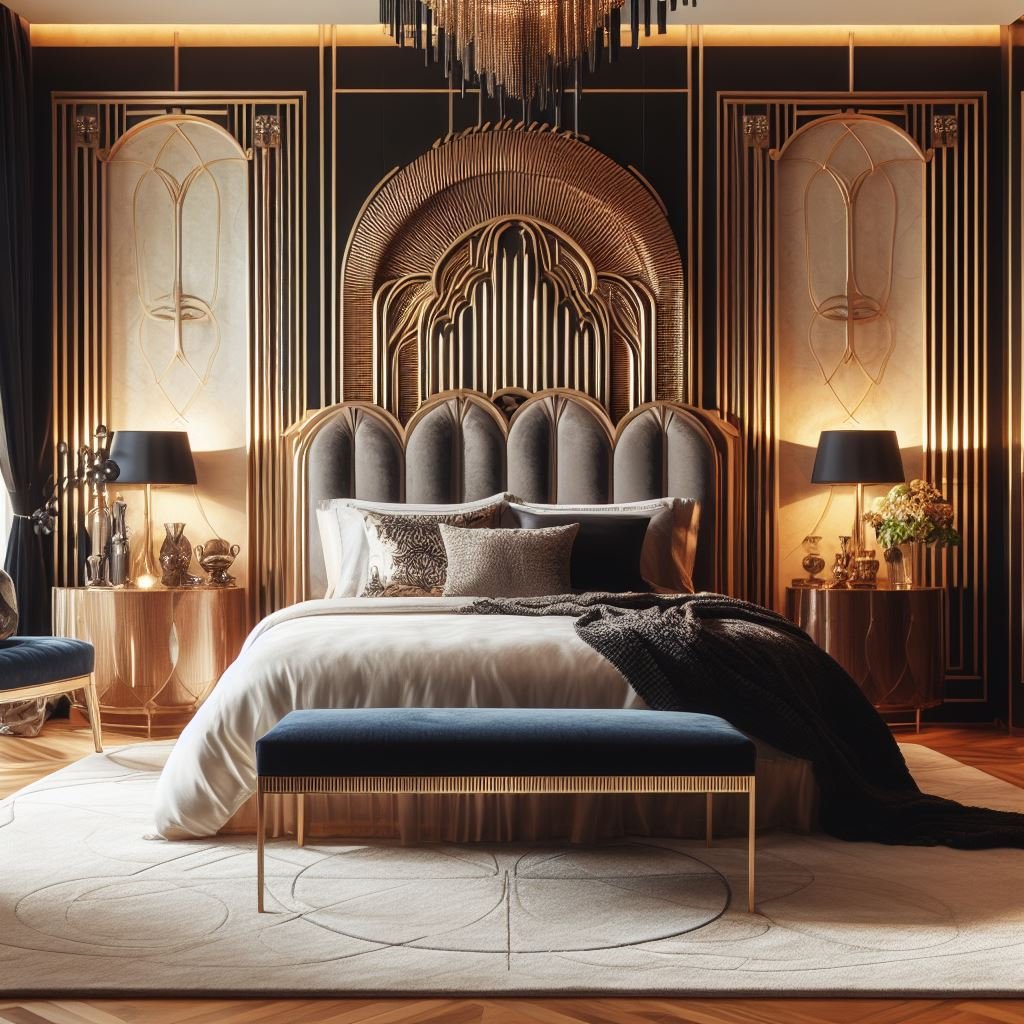The image showcases a high-class, elegantly appointed bedroom that exudes a Great Gatsby era vibe, reminiscent of the 1920s and 1930s. Central to the room is a large bed with a long, rounded headboard adorned with decorative pillows. The bed is dressed in a white comforter with a black blanket casually draped, revealing a white mattress that extends to the floor. Below the bed sits a gold-legged black cushioned stool. A square white rug lies beneath the bed, and on either side of the bed are tables draped in long silky cloths, each supporting a black lamp with gold trim and black lampshades. The walls are a tan hue, adorned with golden brass features and inlaid pipes. On the left side of the room is a plush black chair with gold or tan accents. Overhead, a chandelier, a blend of black and gold, illuminates the room, adding to its opulent atmosphere.